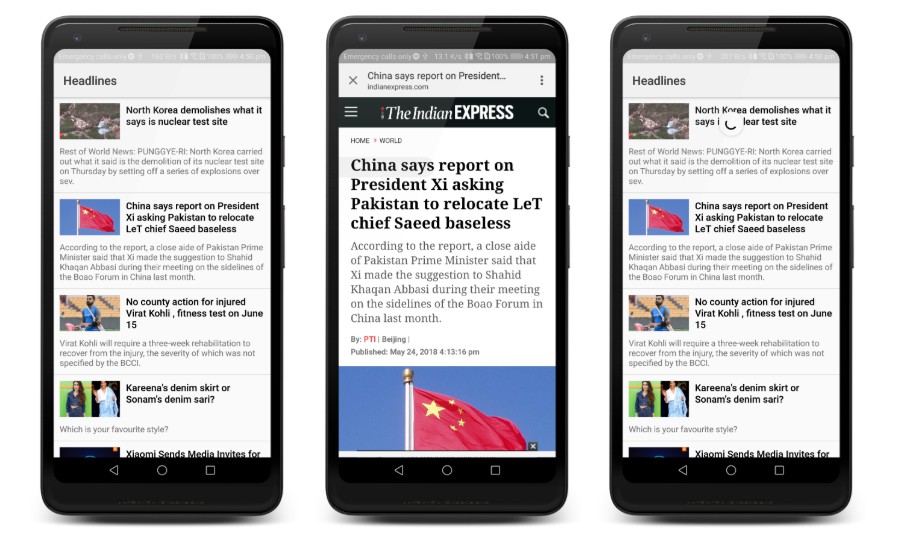This photograph captures three cellphones lined up horizontally, each displaying different pages from the same website. The cellphones are spaced apart, providing a clear view of the content on each screen.

- **First Screen:** The cellphone on the far left displays the "Headlines" section. There are four distinct articles, each featuring a photo thumbnail on the left side. To the right of each thumbnail, the article's headline is prominently shown in bold black font. Beneath each headline, there is a brief excerpt summarizing the story.
  
- **Second Screen:** The middle cellphone features a different page. At the top, there is a noticeable pop-up with an ‘X’ button on the left corner and a menu button on the right corner. Below this pop-up, the title of the website, "The Indian Express," is displayed. The remainder of the screen contains a full-length article, offering an in-depth read.
  
- **Third Screen:** The cellphone on the far right shows a page identical to the first, labeled "Headlines." Similar to the first screen, it includes four articles, each accompanied by a photo thumbnail on the left, a bold black headline on the right, and a short excerpt below. The layout and design exactly mirror those of the first screen.

This detailed arrangement provides a comprehensive look at the various sections and design elements of "The Indian Express" website as viewed on mobile devices.